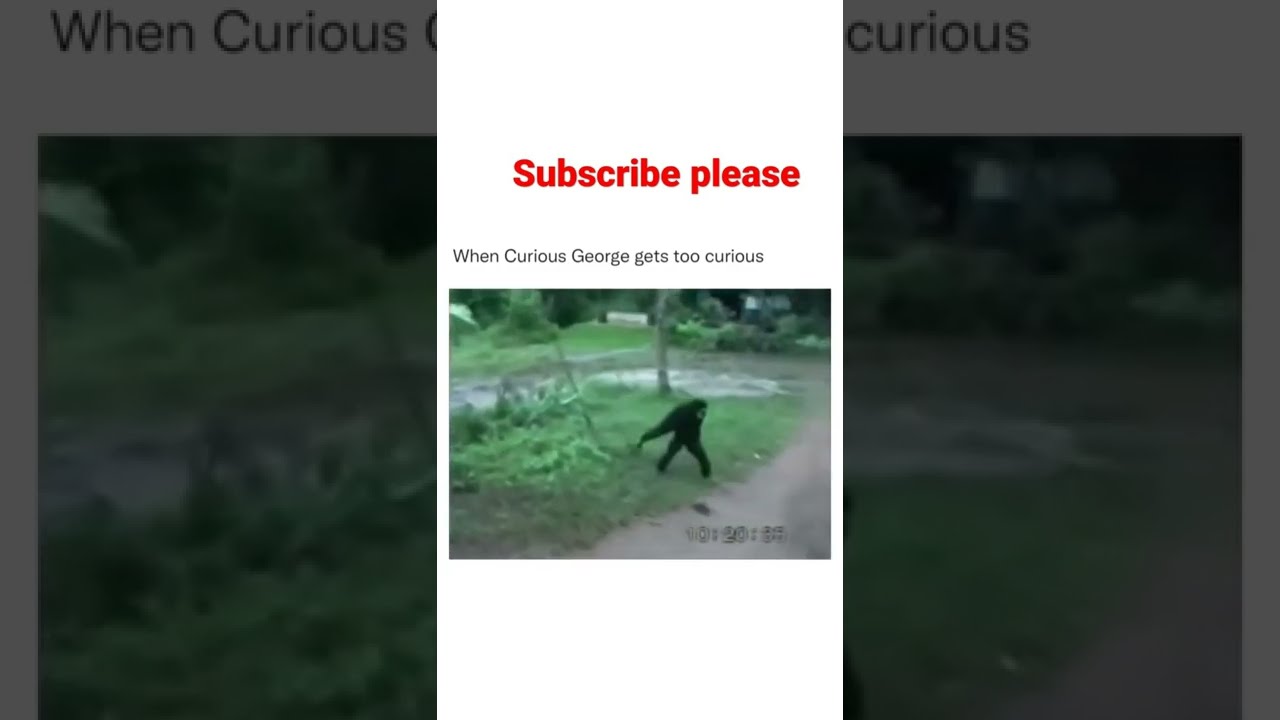The image is a YouTube channel screenshot featuring a thumbnail of a video overlaid on a blurred background version of the same screenshot. The central thumbnail shows a small black-furred monkey walking across a forest path, with typical colors of green from the trees and light brown from the dirt, indicating it's an outdoor forest setting. The detailed environment also includes a small river or stream nearby. Positioned above the thumbnail, bold black text reads, "When Curious George Gets Too Curious," while red text above that encourages viewers with "Subscribe Please." In the bottom right corner of the thumbnail, a timestamp of 10:20 is visible, further emphasizing the candid nature of this security camera footage-inspired scene.